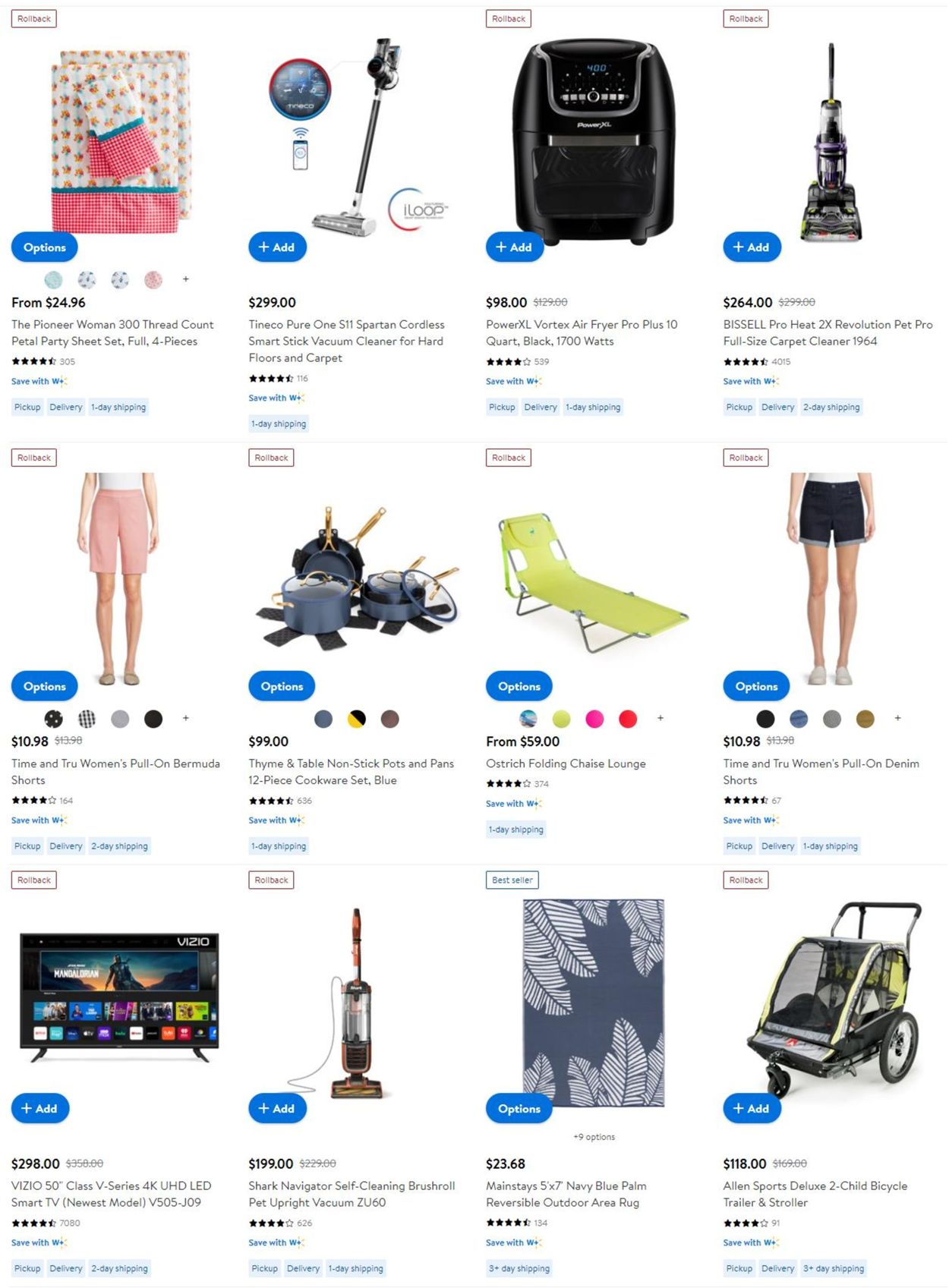The image shows a selection of products from the Walmart online store, arranged in a grid of four items across and three rows down. In the top left corner, there's a discounted product marked with a "rollback" label: the Pioneer Woman 300 Thread Count Petal Party Sheet Set, which is depicted in an image resembling napkins adorned with orange-colored vegetables or fruits. This set is priced at $24.96. To its right, there's a Smart Stick Vacuum priced at $299. Next in line is a Power XL Vortex Air Fryer for $98. The final product in the first row is a ProHeat 2X Revolution Pet Pro Carpet Cleaner, available for $264.

In the second row, the first item from the left is a pair of pink shorts priced at $10.98. The next product is a cookware set for $99. Following this, there's a green folding chair priced at $59. The fourth item in the second row is another pair of shorts, this time in denim blue, also priced at $10.98.

The bottom row features a diverse selection: there's a television, a vacuum cleaner, a rug, and a child's bicycle, although the specific prices and detailed descriptions for these items are not provided in the initial voice description.